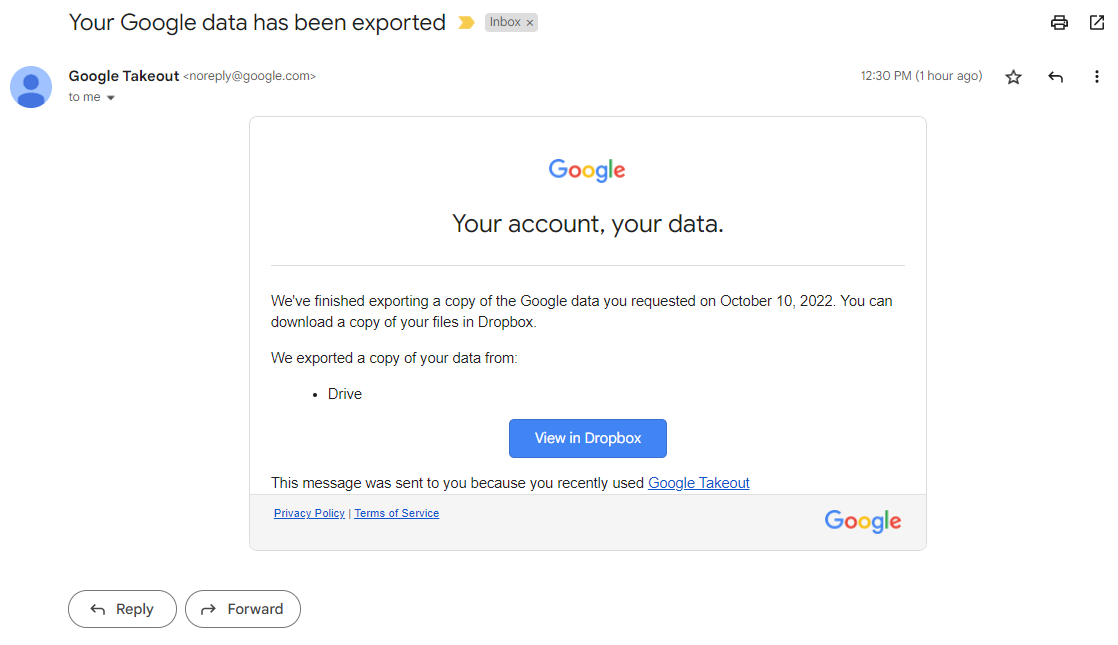A detailed screenshot caption might look like this:

---

The image is a screenshot of an email notification from Google Takeout. At the top of the email, a yellow arrow points to a gray rectangle with the word "Inbox" inside it. On the far right, a printer icon is visible. The email header shows "Google Takeout" on the far left, followed by "No reply at google.com" addressed to the user's email. On the far right, the timestamp reads "12:30 p.m. one hour ago."

In the top navigation bar, there is a star icon, a left-pointing arrow, and three vertical black dots representing an options menu.

The main body of the email starts with the Google logo and states, "Your account, your data." It informs, "We finished exporting a copy of the Google data you requested on October 10th, 2022." The user is instructed, "You can download a copy of your files in Dropbox," followed by the line, "We exported a copy of your data from Drive."

A prominent blue rectangle labeled "View in Dropbox" in white letters provides a call-to-action button for the user. Below this button, additional information explains that the message was sent to the user because they recently used Google Takeout. There are links to the Privacy Policy and Terms of Service.

At the bottom right corner of the email, the Google logo appears. The bottom left corner displays the options "Reply" with a left-pointing arrow and "Forward" with a right-pointing arrow.

The email is devoid of photographic elements, people, animals, or automobiles. The entire screenshot focuses on the notification regarding the export of Google data via Google Takeout.

---